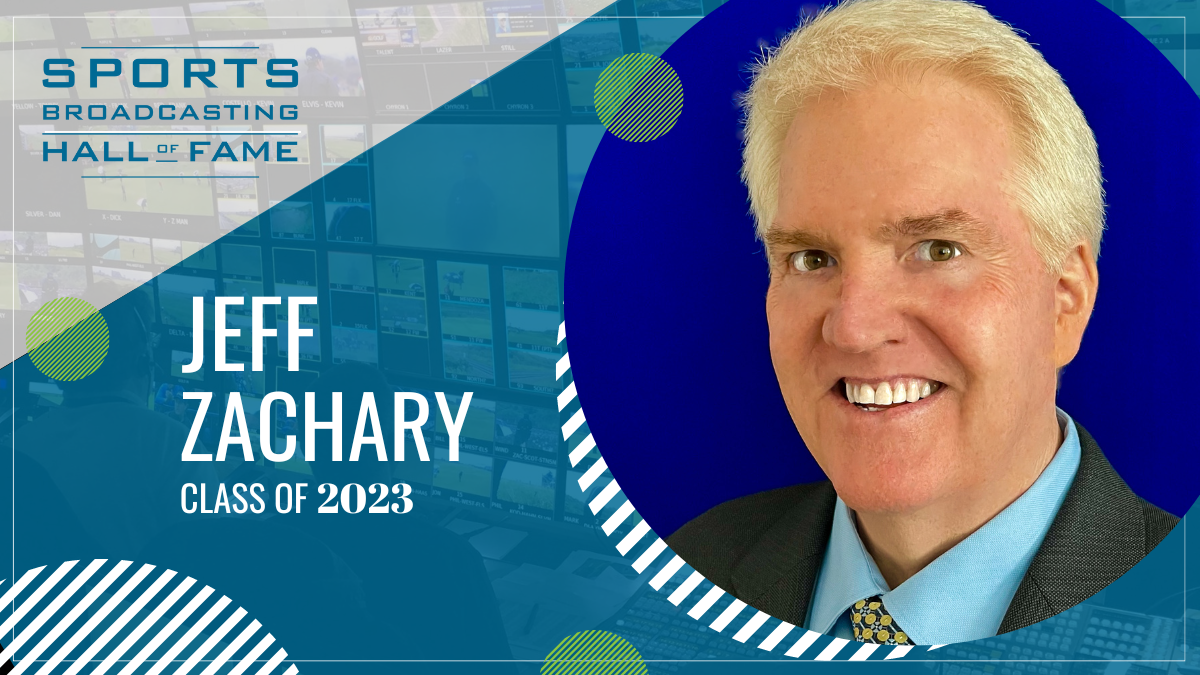This image is a detailed advertisement banner for the Sports Broadcasting Hall of Fame. Featured prominently is Jeff Zachary, Class of 2023. The layout includes blue, gray, and beige colors. In the top left corner, bold blue text reads "Sports Broadcasting Hall of Fame," followed by "Jeff Zachary, Class of 2023." On the right side, there's a circular portrait of Jeff Zachary, an older white man in his 50s or 60s, smiling at the camera. He has blonde hair and is dressed in a blue dress shirt and a gray suit jacket. The background features a typical sports broadcasting station with multiple screens displaying various videos. Beneath the text, geometric shapes, including striped circles and blue and gray transparent layers, add a modern touch to the design.